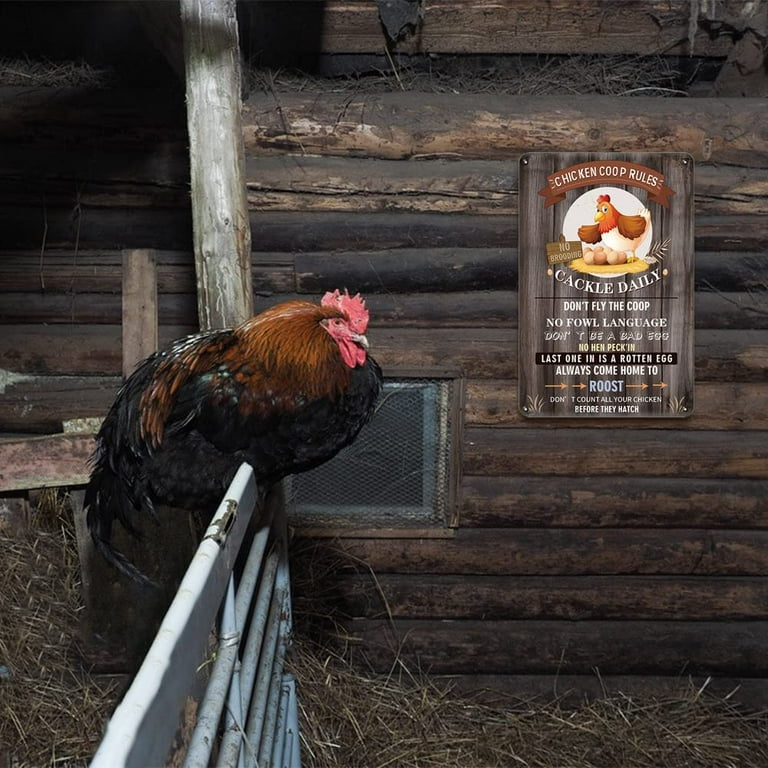This detailed image captures the inside of a rustic, log cabin-style chicken coop with brown wooden slats. The coop floor is strewn with hay, contributing to the rustic charm. A silver-colored fence runs along the left side, and perched on the fence is a real rooster, featuring long brown and black feathers with a distinctive red comb and wattle. Its beak is prominently visible, and it presents a majestic and attentive demeanor.

On the back wall of the coop, directly to the right of a screen door, is a sign titled "Chicken Coop Rules," which adds a whimsical touch to the scene. This sign contains a cartoon drawing of a rooster and several eggs, along with a list of witty rules in white font: "Cackle daily," "Don't fly the coop," "No foul language," "Don't be a bad egg," "Last one in is a rotten egg," "Always come home to roost," and "Don't count the chickens before they hatch." The overall ambiance of the coop is cozy and rustic, with a clear emphasis on both functionality and charm.